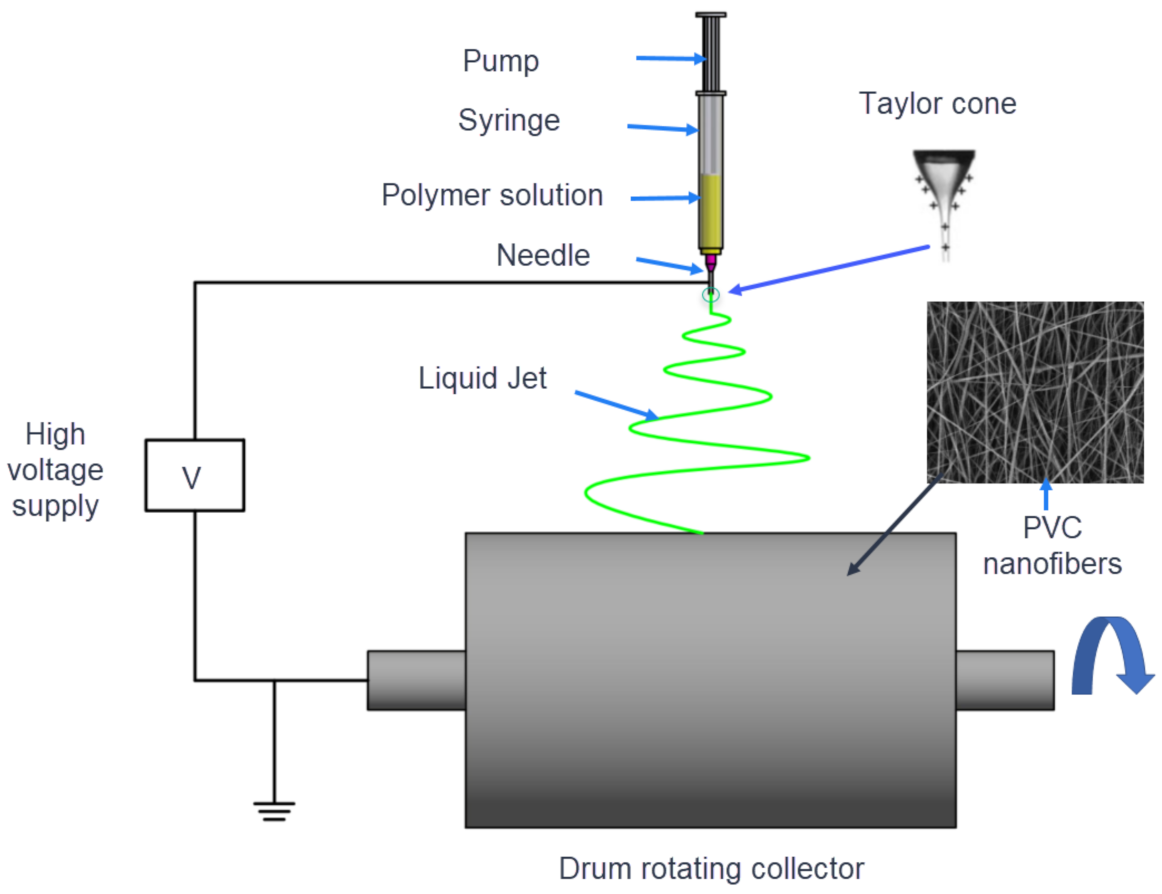The image is a detailed schematic of a system used to create PVC nanofibers. Starting from the left, the process begins with a syringe containing a yellow polymer solution, which is injected through a needle into the system. The needle emits a liquid jet, depicted with wavy green lines and labeled as "Liquid Jet." This jet forms a Taylor cone, a crucial element in the process, illustrated in the top right corner of the diagram. 

As the polymer solution exits the needle, it is combined with a high-voltage supply, indicated by markings of positive and negative charges around the Taylor cone and a box labeled "High Voltage." The high voltage facilitates the formation of the polymer into nanofibers. Subsequently, the liquid jet enters a drum rotating collector, represented by a gray box with blue arrows denoting its rotational motion.

The final product, PVC nanofibers, is shown emerging from the other end of the drum rotating collector, with gray crisscrossing lines on a black background symbolizing the fibers. The entire process is visually enriched by various colors, including blues, greens, yellows, grays, blacks, and whites, adding depth and clarity to the schematic.